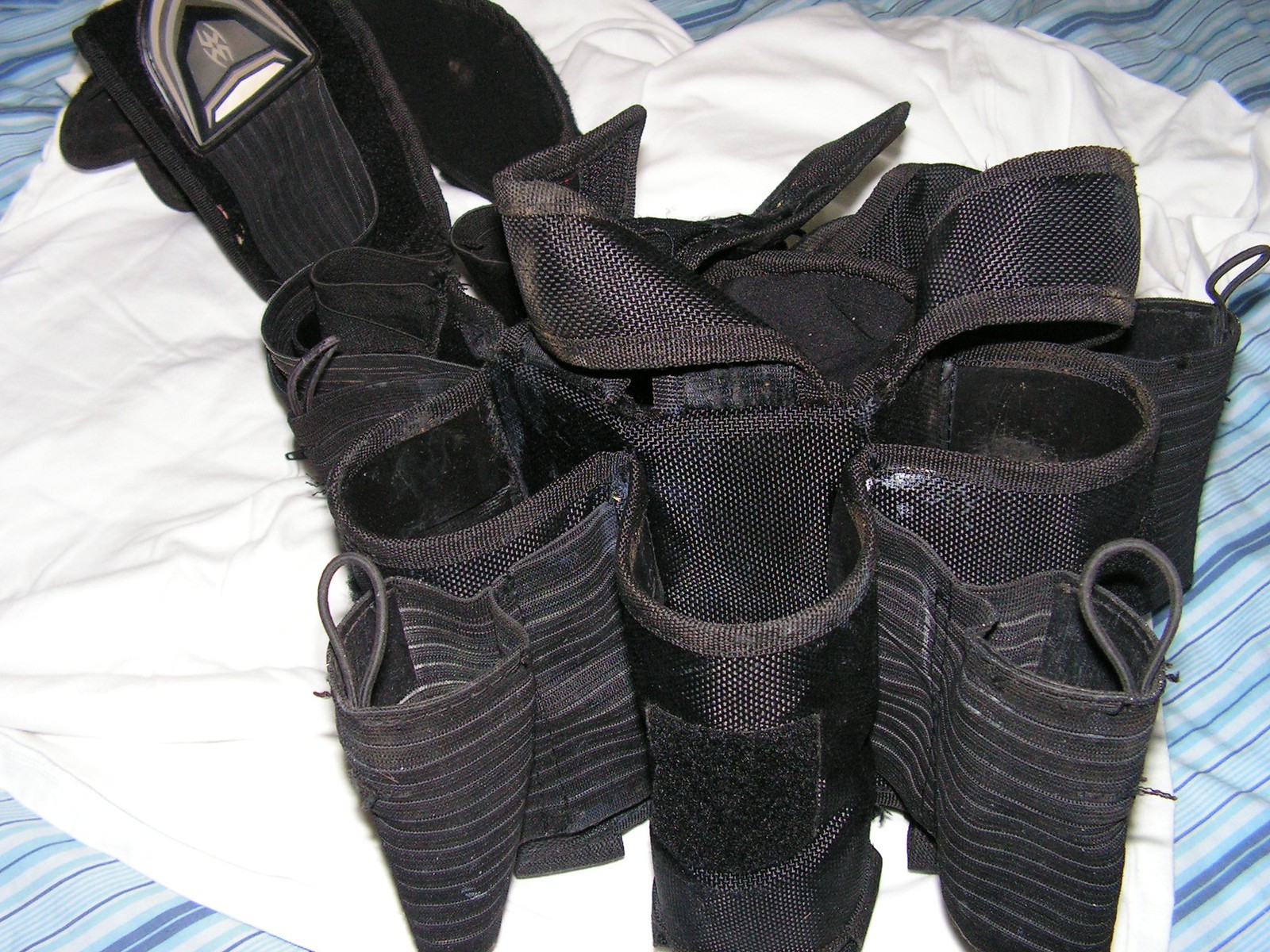This photograph features a black fabric contraption that resembles a durable tool holder, possibly designed for construction workers or for organizing tools around a bucket. The black material is robust and includes multiple compartments, loops, and closures, some secured with Velcro or hooks, ideal for storing various tools or small items. The central section has a round hole, and the entire contraption is arranged in a flower-like pattern. Additionally, there’s a distinct compartment with a beige and brown patch, suggesting the possibility of holding a knife or similar tool. The setup is laid atop a white article of clothing, likely a shirt, on blue and white striped sheets, enhancing the contrast and visibility of the black tool holder.